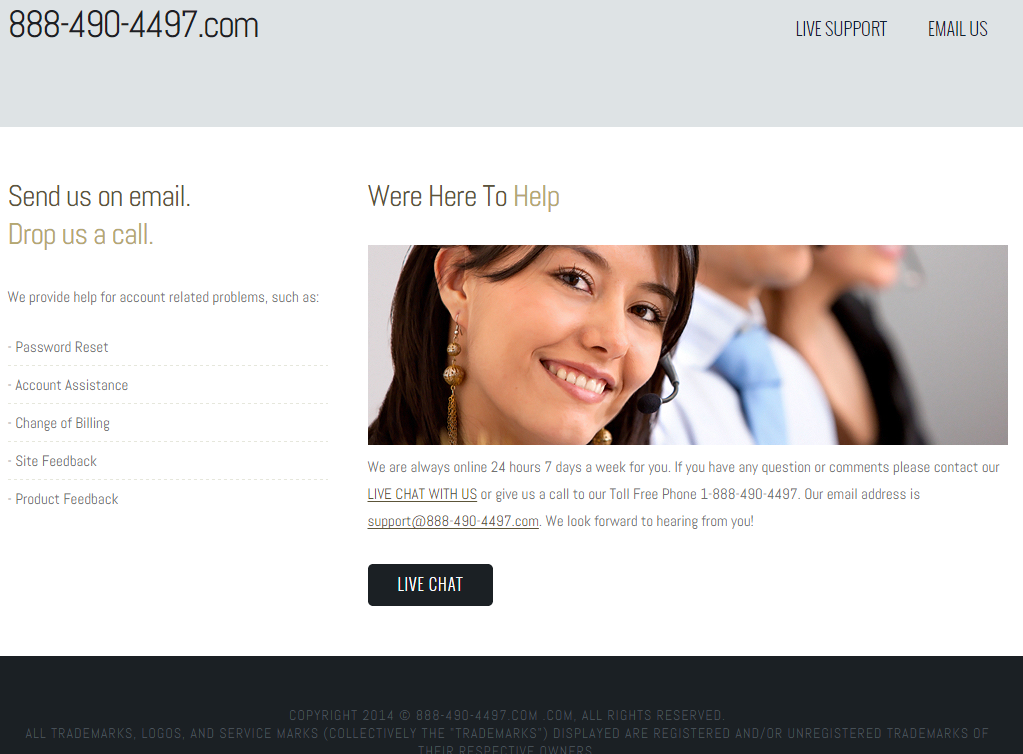At the top of the image, there is a long gray rectangle that features the phone number "888-490-4497" in black text on the left, followed by ".com." To the right of this, there are clickable options labeled "Live Support" and "Email Us." Below this section, on the left side, there is a message that reads: "Send us an email or drop us a call. We provide help for account-related problems such as password reset, account assistance, change of billing, site feedback, and product feedback."

On the right side, the phrase "We're here to help" is prominently displayed. The main part of the image shows a smiling woman with dark eyes, dark hair, and long dangly earrings. Behind her are two figures, visible from the chin and upper chest area. One is wearing a suit and tie, the other is in a black shirt, and both have microphones attached, indicating they are ready to assist.

The image includes a message stating: "We are always online, 24 hours a day, seven days a week. If you have any questions or comments, please contact us." Underneath this message, the phrases "Live chat with us" and "Give us a call at our toll-free number, 1-888-490-4497" are underlined. The provided email address for support is "support@888-490-4497.com."

Finally, at the bottom of the image, there is a black box with the words "Live Chat" written inside.